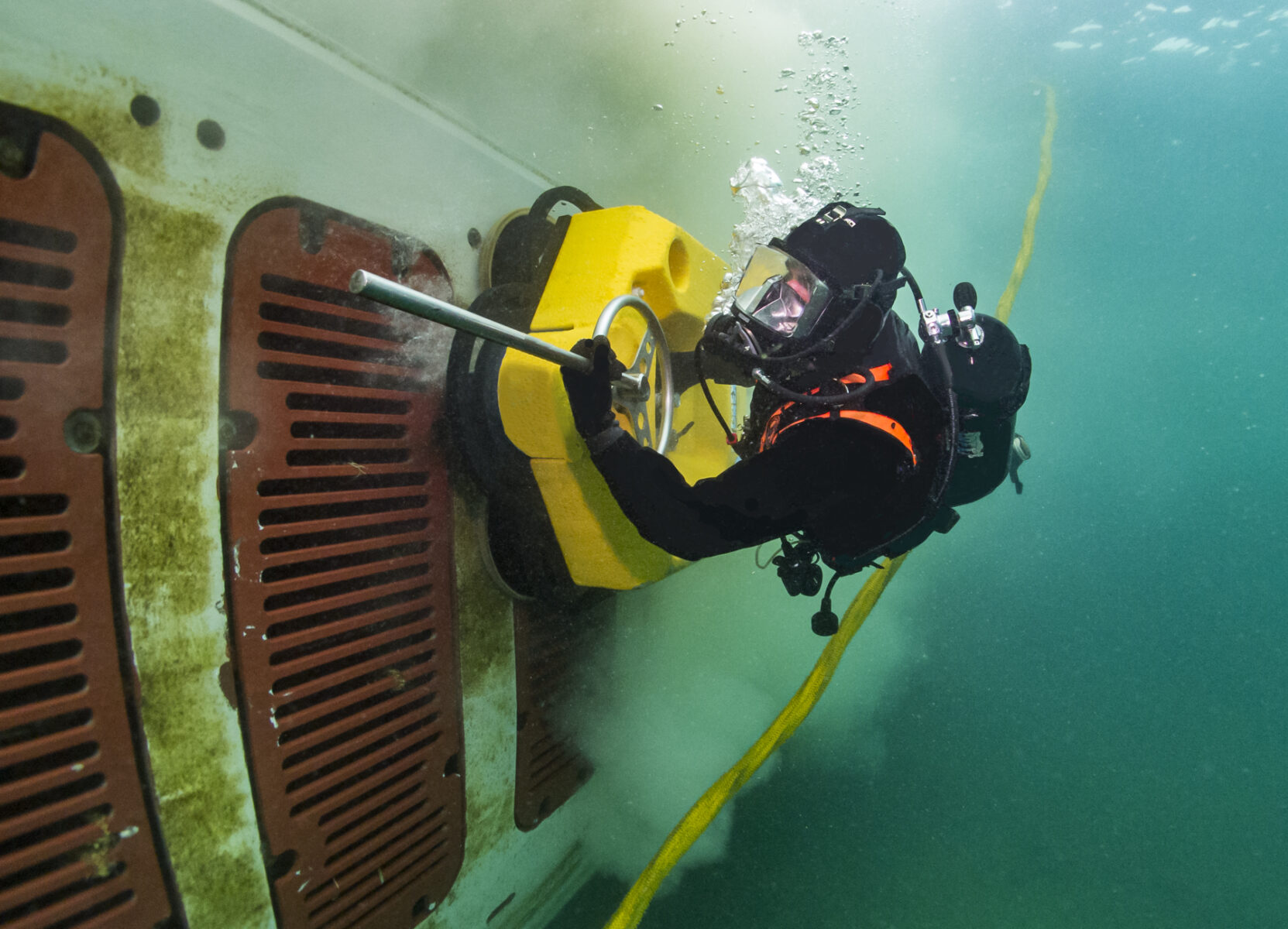The image depicts a scuba diver, clad in a black wetsuit with orange straps crossing his shoulders, working underwater. The photo is oriented sideways, giving a horizontal view of the scene. The diver is near a large, white wall that spans from the upper left to the lower right corner of the frame. This wall, which might be part of a boat or a large tank, features brown slotted panels and green moss growing on its surface. The diver is holding a yellow cleaning device with a silver steering wheel and a protruding metal rod in his left hand. Bubbles can be seen streaming out of his breathing equipment and the cleaning device. Additionally, a long yellow cord extends from the top of the water down to the bottom of the picture, possibly aiding the diver in his underwater task. The entire setting suggests he might be engaged in cleaning or maintaining the surface of a submerged vessel.